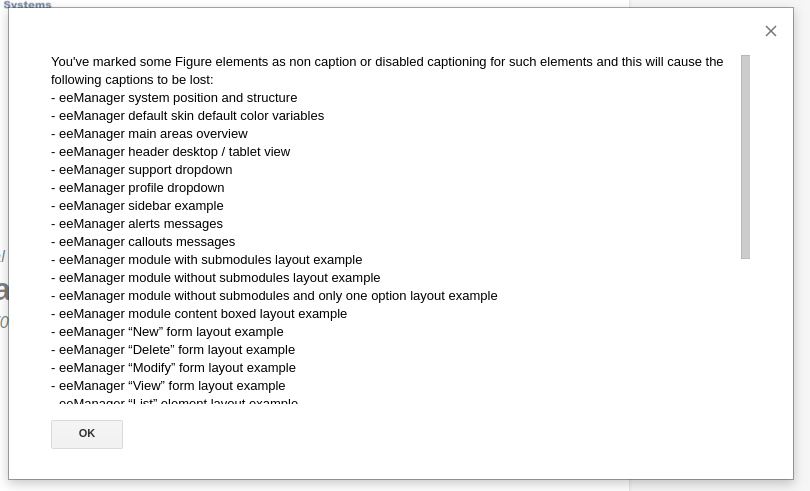An image shows a predominantly gray square, with a more detailed center featuring various elements that appear to relate to a user interface or software application. This central area contains dropdown menus, form layouts, examples of modified forms, and several modules used in managing content. Specific references to management tasks, such as the assistant manager position search and various manager profile options, suggest that the content is likely related to a project management or administrative tool. This detailed focus on user interactions highlights aspects like test houses, support jumps, and a myriad of message modules. The top and bottom of the interface display system information and other user options, adding to the functional complexity of the window.